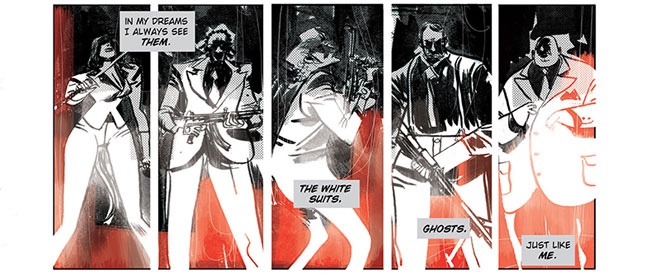The image is a five-panel cartoon rendered in black, white, and red, featuring distinct characters in a noir style. All the characters are either partially or fully dressed in white suits, contrasting sharply with the vivid red backgrounds and black-shadowed details.

In the first panel, a woman in a white suit is seen holding a sword; her face partially obscured by shadows, with her knees bent towards each other in a crouched stance. The top left of this panel contains a text bubble that reads, "In my dreams I always see them."

The second panel introduces a masked man in a white suit and tie, armed with an SMG (submachine gun), standing against a red background like the previous one.

The third panel depicts a side view of a man with curly hair wearing a top hat, also donning a white suit and holding a firearm. Below him, towards the bottom third section of the panel, another text box declares, "The white suits."

In the fourth panel, a man in black overalls with a white shirt is shown holding a gun, with a text box beneath him that reads, "Ghosts."

The final panel features a rotund bald man with a clown-like round nose, dressed in a white suit, white tie, black shirt, and red pants. The last text bubble says, "Just like me."

The recurring theme of the characters all wearing white suits alongside the phrases suggests a haunting self-reflection or a metaphorical link to ghostly apparitions, deepening the sinister and introspective tone of the cartoon.